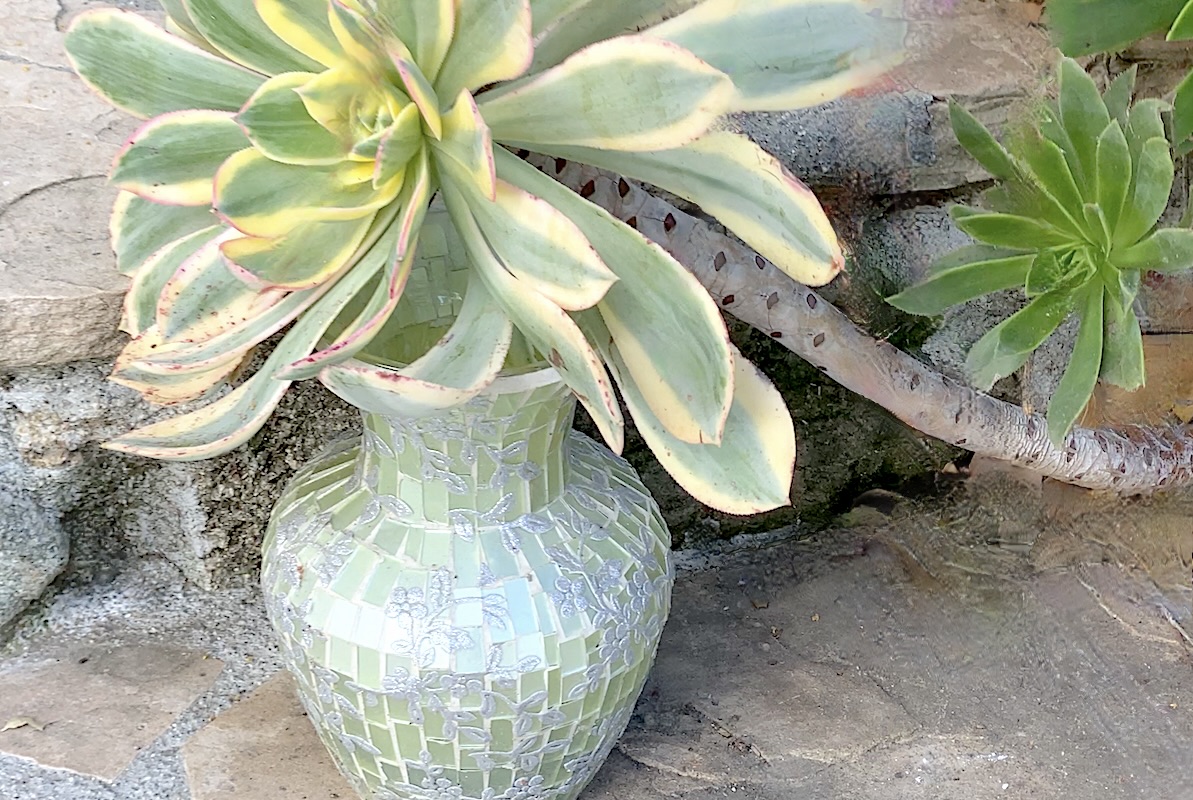In this outdoor photograph, the focus is a large, ornate glass pot situated on a stone pathway with a stone wall in the background. The pot, decorated with leaf motifs and light green in color, appears to have a succulent growing from it. However, upon closer inspection, the succulent is actually sprouting from a large branch positioned directly behind the pot. The succulent's leaves, which are outlined in yellow with hints of red, extend over the pot, creating the illusion that they are growing from within. To the right of the pot, another succulent with deeper green leaves can be seen. The scene is framed by stones and a mix of concrete paving, with some additional greenery visible in the top left corner. This tropical setting is reminiscent of a desert garden, characterized by its vibrant yet resilient plant life.